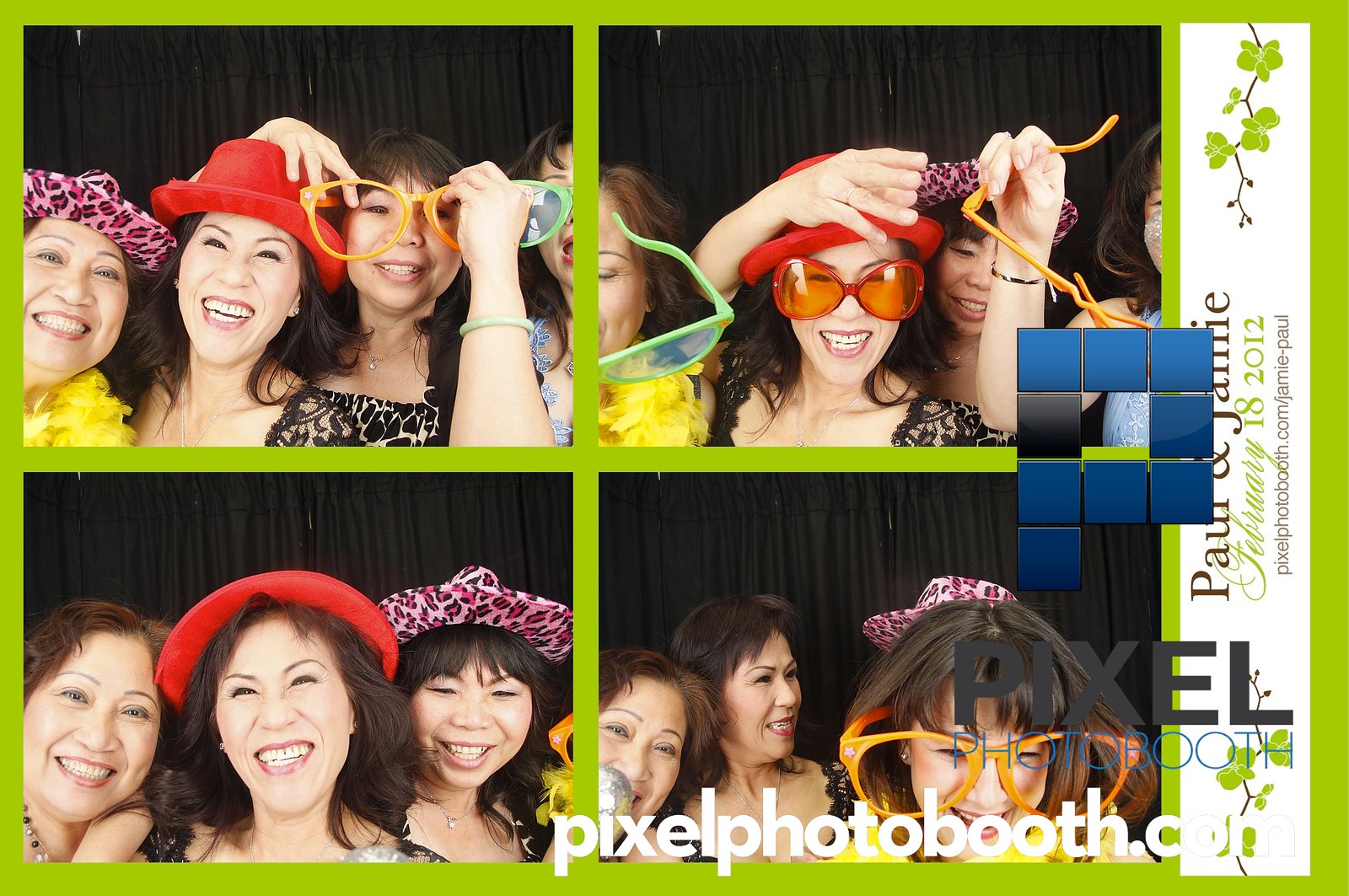This image is a vibrant, green-bordered collage composed of four photographs arranged in a 2x2 grid with playful and jovial scenes. Each photo depicts the same group of four women, all adorned in comically oversized sunglasses and whimsical hats, posing and playing with the props. The photos capture their expressions and interactions from the neck up, highlighting their smiles and laughter. The sequence includes different groups and combinations of the women, creating a lively, dynamic feel to the image.

Overlaying the bottom of the collage, the text "pixelphotobooth.com" is prominently displayed in white. There's also a P-shaped logo comprising blue and black squares that reinforce the branding. The right edge of the collage features a slightly tilted white bar running vertically with the inscription "Paul and Jamie, February 18, 2012," suggesting a personal or celebratory event. The entire collection exudes a cheery atmosphere typical of photo booths found at festive gatherings, such as weddings or parties, emphasizing spontaneous and candid moments.